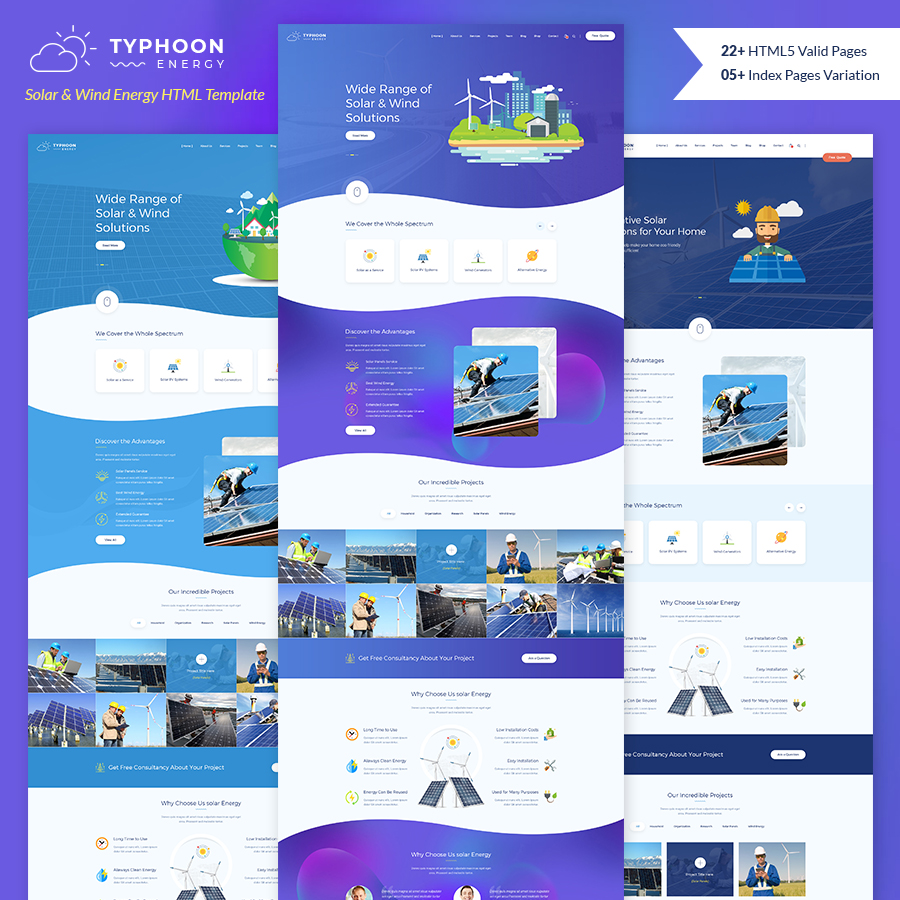This brochure for Typhoon Energy showcases their extensive range of solar and wind energy solutions using an HTML template. Against a teal background, bold text highlights their diverse offerings in solar and wind energy, stating, "Wide Range of Solar and Wind Solutions." A contrasting blue background emphasizes the call to action, "Discover the Advantages."

The brochure features several images: a group of technicians, all equipped with clipboards and computers, are seen analyzing and working on solar panels and wind turbines. The text reiterates their commitment, "We cover the whole spectrum," along with another prompt to "Discover the Advantages."

One image captures a technician physically installing a solar panel on a rooftop, demonstrating their hands-on approach. The brochure also showcases their various impressive projects, illustrating different configurations of solar panels that are not limited to rooftop installations. In another section, lined-up wind turbines are displayed, indicating the scale and organization of their wind energy projects. 

All personnel shown are equipped with hard hats, underscoring their commitment to safety. The brochure invites potential clients to "Get a Free Consultation About Your Project." A somewhat blurred section mentions the reasons for choosing U.S. solar energy and hints at "airtight clean energy," accompanied by an image of two wind turbines and two solar panels, reinforcing their dual focus on solar and wind energy solutions.